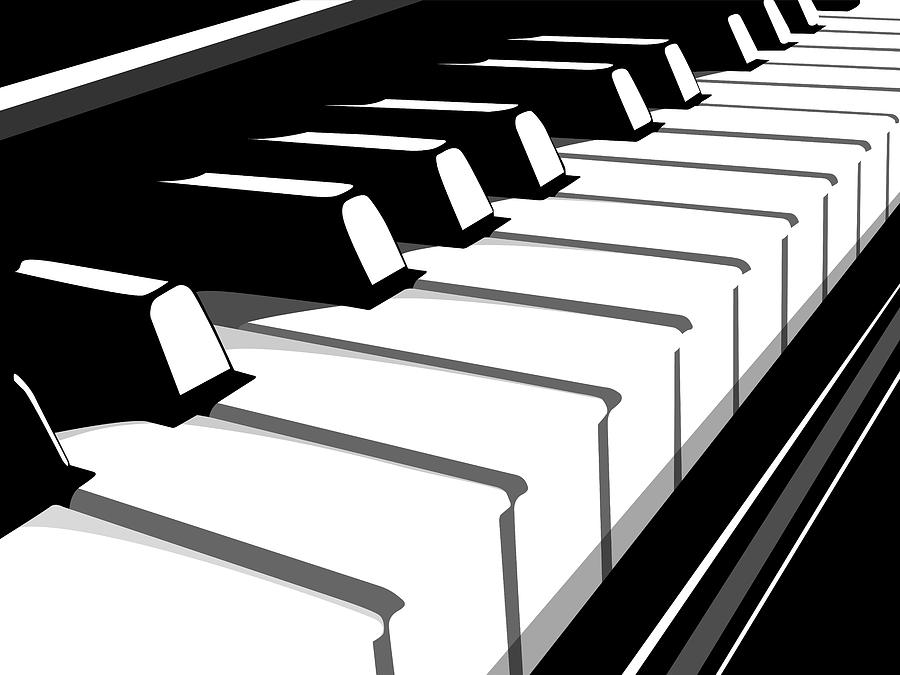This is a detailed, cartoon-like, black and white image of a close-up section of a piano keyboard. The composition prominently features the white ivory keys, set diagonally from the bottom left to the top right of the image, contrasted by the shorter black keys. The visual centers around approximately 15-20 white keys and about 8-9 black keys, with clear outlines in deep black that define the shapes. Notably, the top left and bottom right corners of the image are occupied by black triangular shapes. There is also a reflective quality suggesting a glossy black piano surface beneath the keys, adding depth to the predominantly monochrome palette of the illustration.